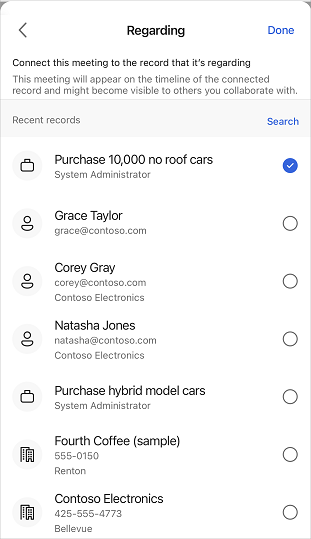"Screenshot of a Bluetooth connection interface displaying various meeting and contact details. The meeting is being recorded and will appear on the timeline of the connected record. The screen shows a recent Bluetooth search indicating the presence of a briefcase with a note to purchase $10,000 worth of cards. Several contacts are listed, including Grace Taylor (Grace@Contoso.com), Corey Gray (Corey@Contoso.com) from Contoso Electronics, and Natasha Jones (Natasha@Contoso.com) also from Contoso Electronics, none of whom are currently checked. The system administrator circle is marked as checked. Additionally, there’s mention of a building labeled 'Contoso Electronics' with the contact number 425-505-4773, also not checked. The image has a white background, with a triangle icon in the top left corner and some gray text."